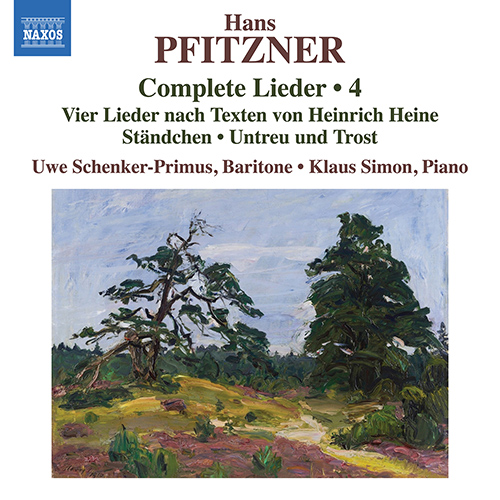The image displays a detailed booklet or page with a white background. In the top left corner, there is a logo inside a blue square box featuring patterned designs with the word "NEXUS" in bold, capital white letters. At the top center, the heading "Hans Pfitzner" is prominently written in large brown fonts. Below this, green text reads "Complete Lieder," and there are German phrases such as "Wir Lieder nach Texten von Heinrich Hein Staunchen, Untrue und Toast." Further down, brown text mentions "Uwe Schenker Primos, Baritone Klaus Simon Piano."

The lower part of the image showcases a painting of a serene landscape, possibly done in oil. It depicts a blue sky and an area filled with greenery, including trees, green grass, and patches of brown soil with small plants. Two main trees are visible in the painting: an evergreen with a traditional conic shape on the right, and a nearly leafless tree with a sparse, skeletal appearance on the left. The ground is varied, with reddish-brown and olive-green or yellow patches, and a line of trees can be seen in the background, contributing to the overall harmony of the scenic view.